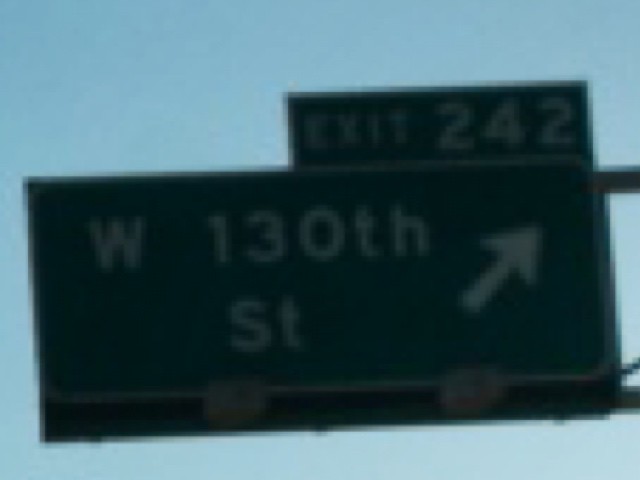The image captures an outdoor scene dominated by a large overhead green highway street sign set against a medium to darker blue sky. The sign, rectangular in shape, is framed by a thin white border and supported by metal rods on the top and bottom. There are two sections: the larger bottom section reads "W 130th Street" with a diagonally upward right-pointing arrow, while the smaller top section reads "Exit 242." The image appears cropped from a larger photo and is slightly grainy and pixelated, but the text is still discernible.